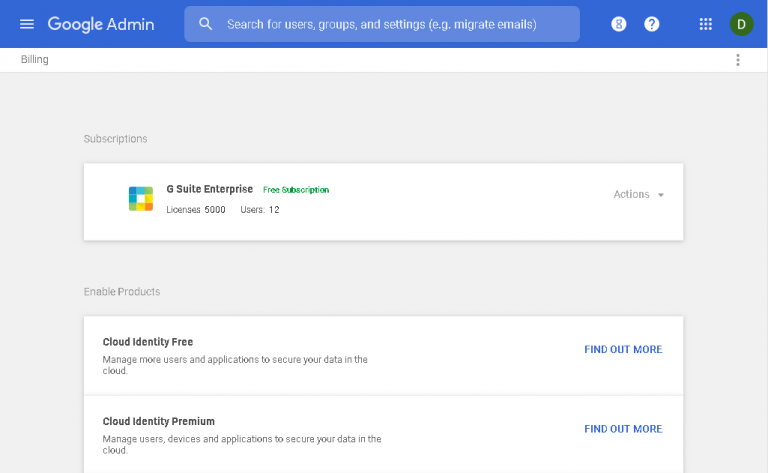This screenshot from the Google Admin console focuses on the billing section. The top of the interface features a blue header containing the Google Admin logo, a search bar for finding users, groups, and settings, along with icons for help, notifications, and account settings. The profile icon is marked with the letter "D."

Below the header, there is a detailed subscription display for G Suite Enterprise. This subscription is labeled as a free subscription, showing that there are 5,000 licenses available, with 12 users currently utilizing them. To the right of this information, there is a drop-down menu labeled "Actions."

Further down, there is a section titled "Enable Products" that offers two options: Cloud Identity Free and Cloud Identity Premium. Each option includes a "Find Out More" link. Cloud Identity Free is designed to help manage users and applications while securing data in the cloud. Cloud Identity Premium provides a more advanced version of the same service, offering additional features, although specific details about these features are not provided in this screenshot. 

In summary, the image captures a comprehensive view of the billing section for a G Suite Enterprise subscription within the Google Admin console, highlighting available licenses, current users, and additional product options.